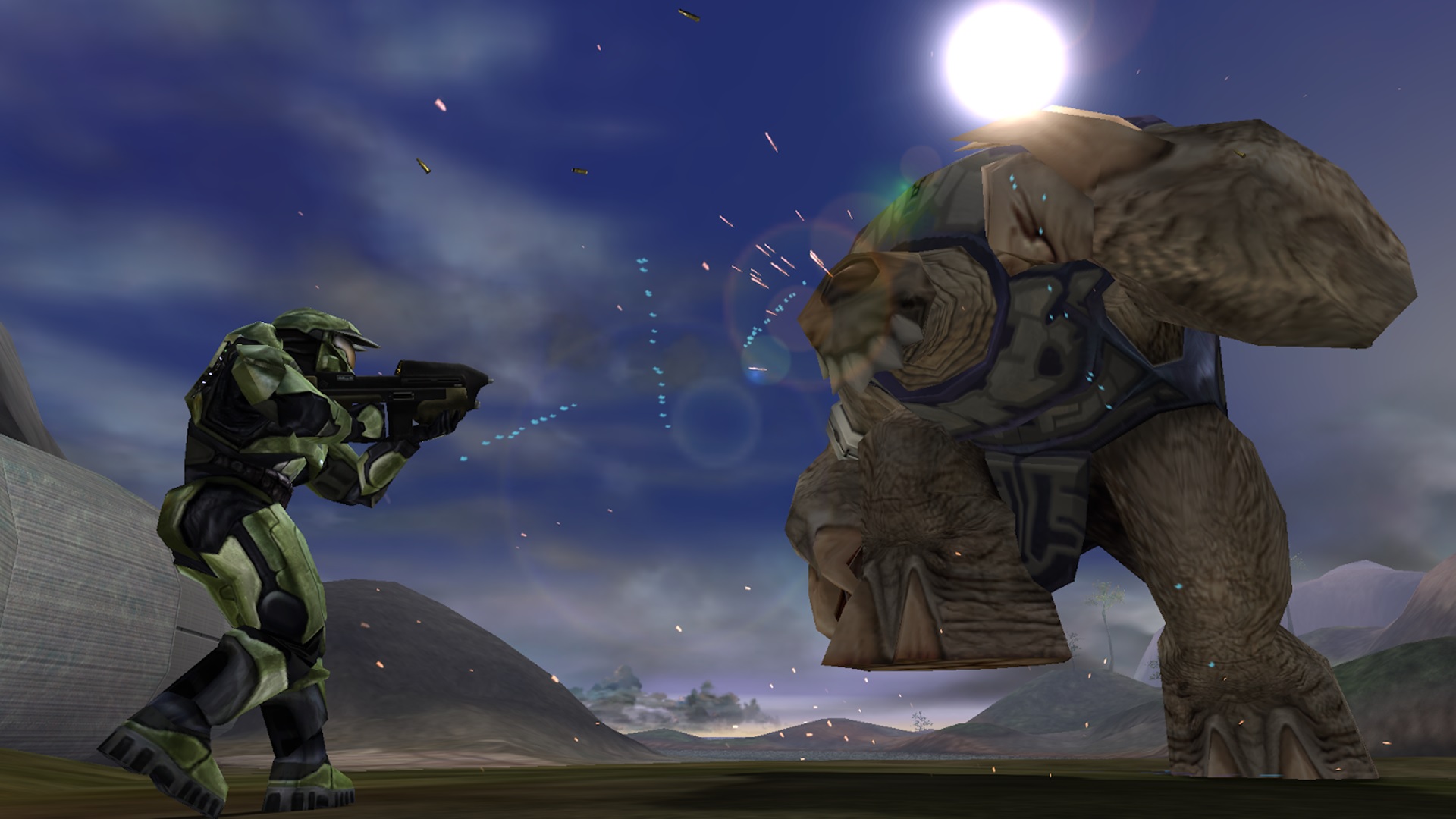This detailed video game image from the Halo franchise captures an intense moment where Master Chief, the iconic future soldier, confronts a formidable rock monster. Master Chief, clad in his signature heavy-duty green armor and helmet with a distinctive green and orange visor, is positioned in the foreground towards the bottom left. He is seen aiming his assault weapon directly at the charging bipedal monster, which is predominantly brown, resembling a fusion of tree stumps with stubby teeth and large paws with big nails. The scene unfolds in a desolate, barren wasteland with sandy hills and a nearby bunker hinted in the background. The atmosphere is set under a clear night sky illuminated by a full, shiny white moon, casting a stark lunar glow over the unfolding battle.